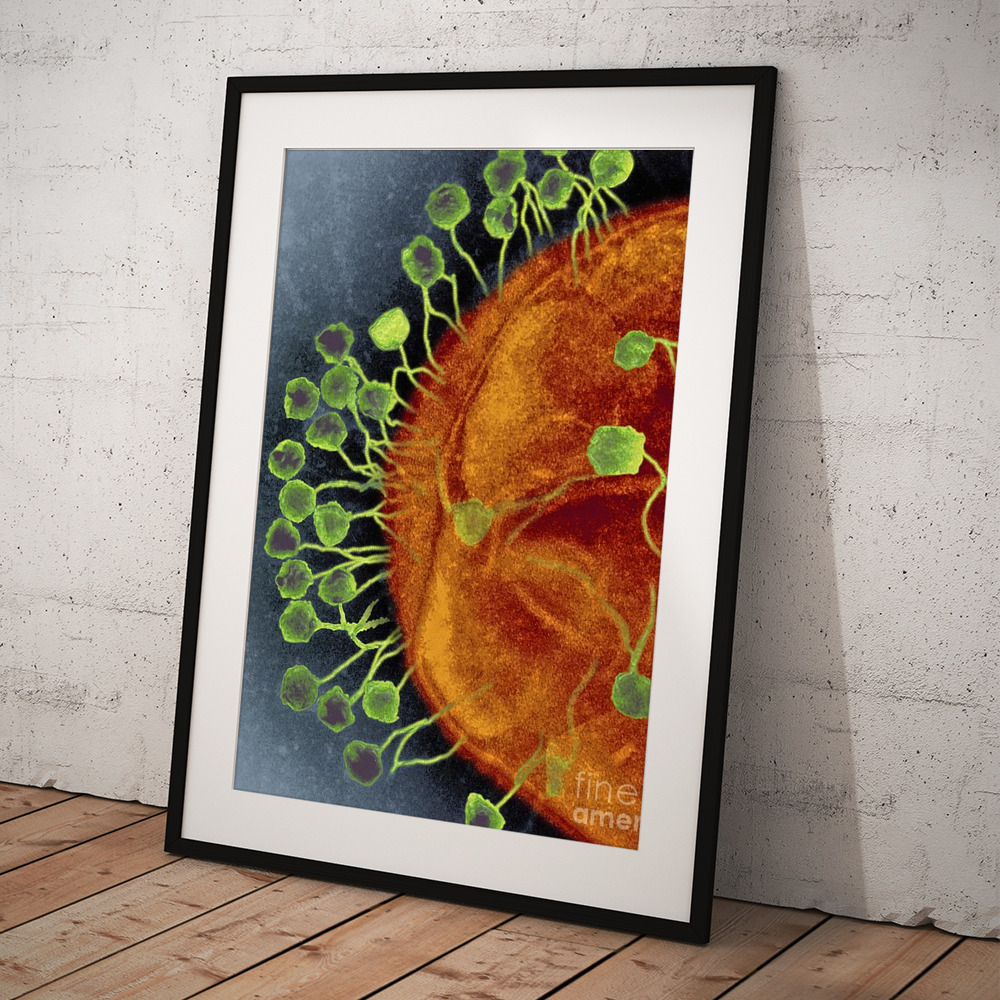The image depicts a vertical rectangular framed picture leaning against a somewhat dirty and unfinished gray wall, possibly a display panel. The floor is composed of rough, unfinished hardwood planks. The frame of the picture is black with white matting. Within the frame, the artwork features a large brown half-circle, reminiscent of either a planet or a seed, with numerous green sprouts or thin lines emerging from it, set against a blue-black background. The overall impression is that of life or growth emanating from a central organic form.